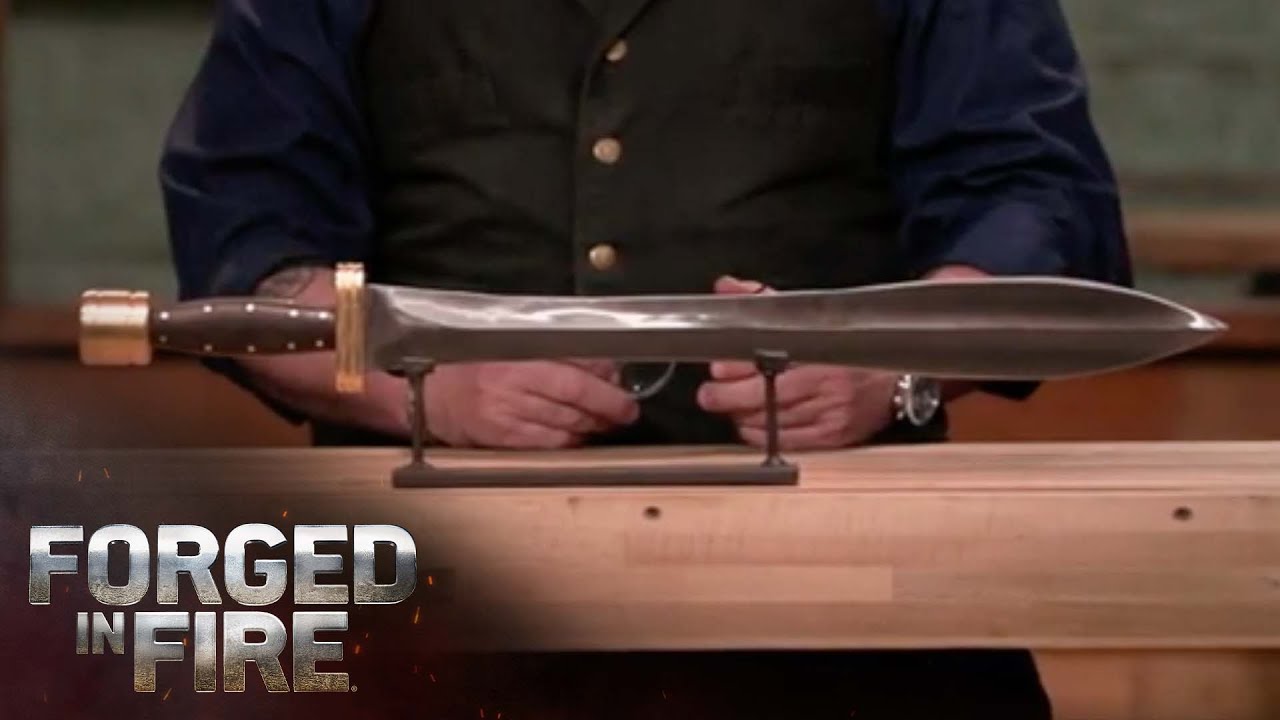The image displays a sword prominently positioned on a light brown wooden table. The sword, which has a dark brown handle adorned with gold dots, features a golden butt and guard. Its blade is a striking silver color, narrowing and then broadening before coming to a point. The sword rests securely in a brown stand with two upturned arms, which holds it in place.

Behind the table stands a man, of whom only the midsection is visible. He has light skin and wears a black button-up shirt with blue sleeves ending at the elbows. The shirt has three golden buttons down the center. His forearms, which rest on the wooden surface, reveal a tattoo on his upper right arm and a wristwatch. His black pants are also visible. 

The background is gray, offering a neutral contrast to the scene. At the bottom left corner, the bold silver text "Forged in Fire" appears, indicating a connection to the TV show known for its blacksmithing competitions. The image quality is slightly blurred, suggesting it may be a screen capture from the show.